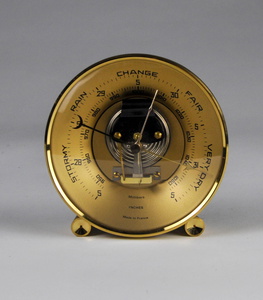The photograph features a barometer that resembles a round clock, set against a background that transitions from shadowy gray at the top to a bright white at the bottom. The barometer, composed of yellowy gold metal with black lettering, dominates the center of the image. It is designed to sit on a table, supported by two small gold pieces. The face of the barometer is detailed with words indicating different weather conditions—'stormy' at approximately 8 o'clock, 'rain' at 10 o'clock, 'change' at 12 o'clock, 'fair' at 2 o'clock, and 'very dry' at 4 o'clock. It features two or three dials with additional numbers arranged in a circle, and a central black metal piece that secures the needles. There is some small, unreadable text at the bottom of the barometer.